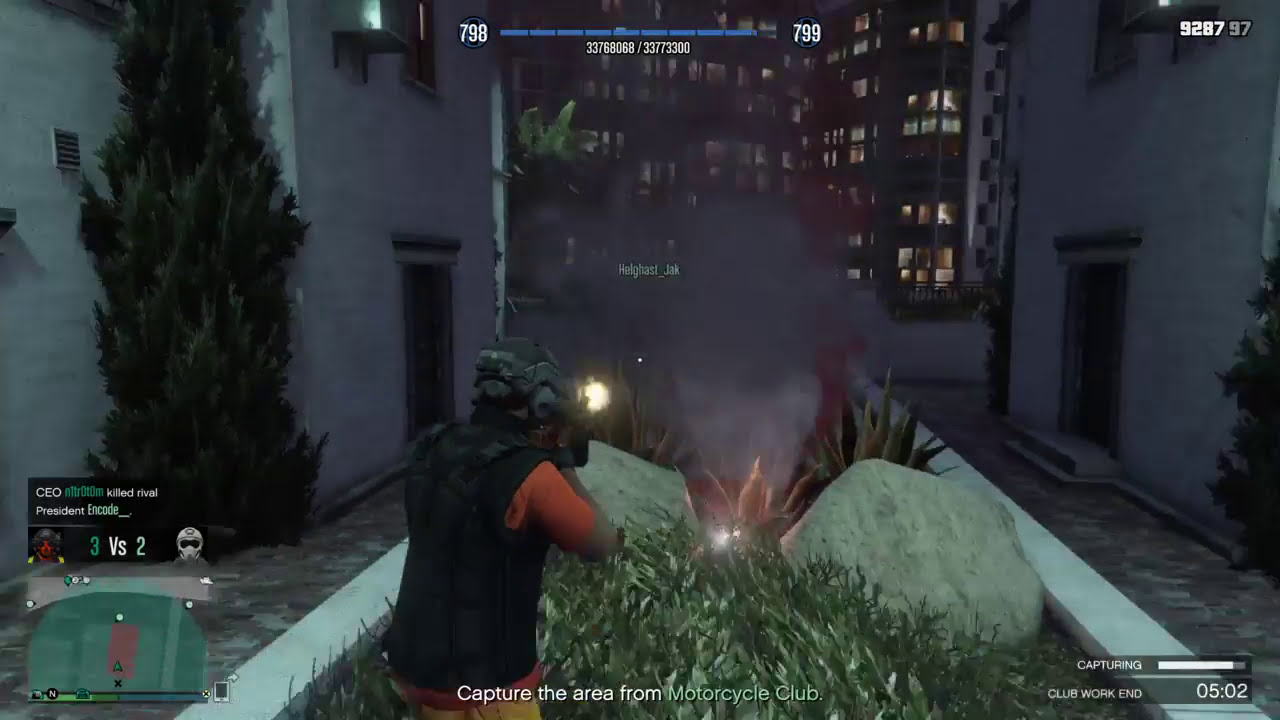The image is a detailed screenshot from Grand Theft Auto, showcasing a nighttime scene in a courtyard between two white apartment buildings. The main character, who is central to the action, is depicted wearing a black bulletproof vest over an orange short-sleeve shirt, with a camouflage helmet and what appear to be ear guards. He is actively firing his weapon amidst the chaos. Smoke from a recently detonated flashbang grenade rises near him, adding to the intensity of the scene. The surrounding area features plants in a concrete structure and has visible grass and rocks in front of the character. The sky is dark, and silhouettes of distant buildings with lighted windows contribute to the ambiance. In the foreground, gameplay HUD elements indicate the objective "capture the area from Motorcycle Club" with a mini-map and enemy indicators on the bottom left. The progress bar and a five-minute, two-second timer at the bottom right demonstrate the capturing process, along with a score count of 3 vs 2. The player's level is denoted as 799, and the ammo count on the top right reads 9287/97. Overall, the intricate details and HUD features authentically convey the tense atmosphere of a high-stakes mission in the game.